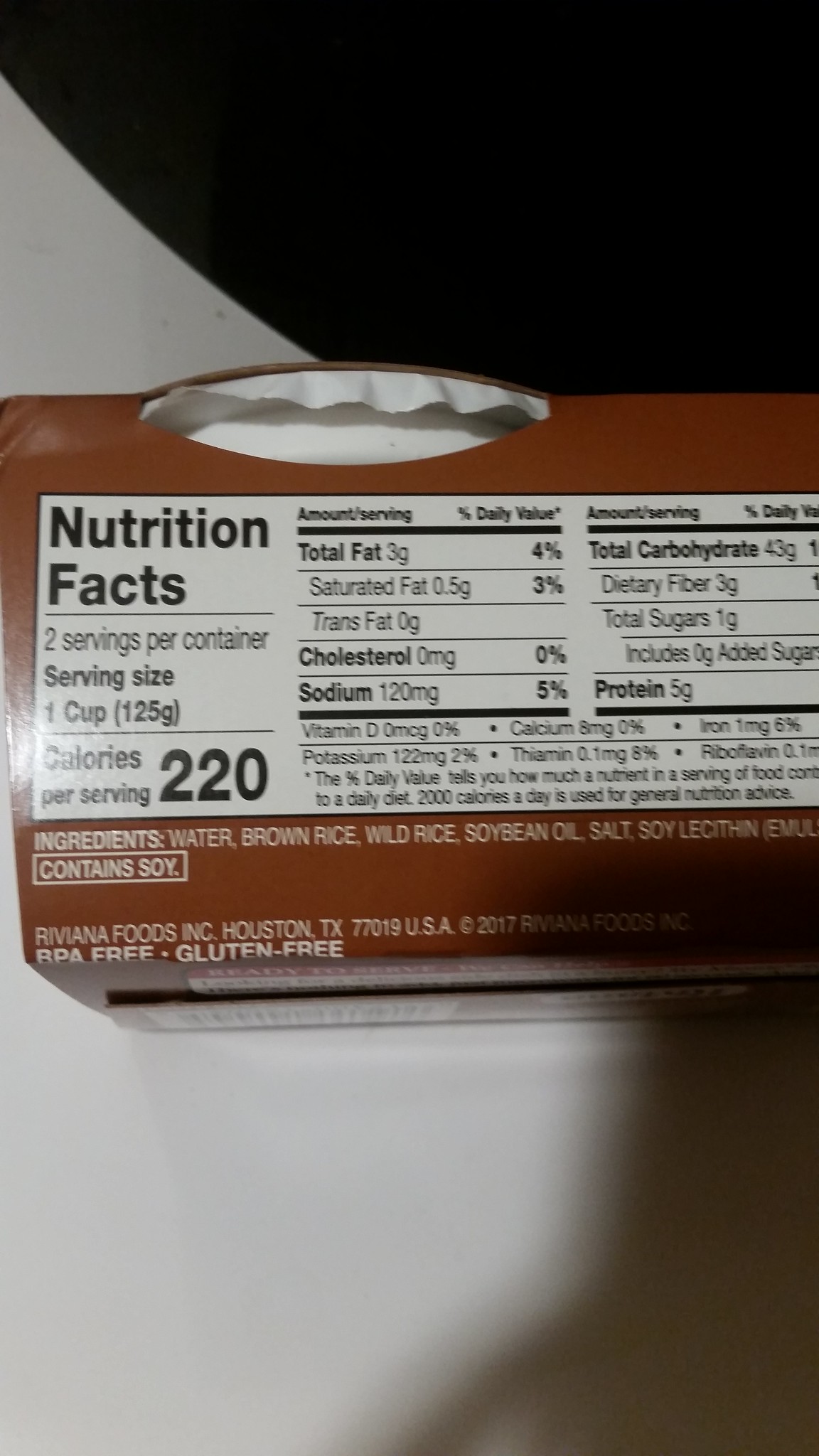This color photograph features a detailed view of the nutritional label on what appears to be the side or top of a brown cardboard food package. At the upper part of the box, a white foil jar or container peeks out through a slit. In the top right corner, there's a black area in the background. The nutrition label itself is white with black text, listing detailed nutritional information per serving. Each serving is one cup, weighing 125 grams, with two servings per container. Nutritional specifics include 220 calories, 3 grams of total fat (4% DV), 0.5 grams of saturated fat (3% DV), 0 grams of trans fat, 0 milligrams of cholesterol, 120 milligrams of sodium (5% DV), 43 grams of total carbohydrates, and 5 grams of protein. Below the main nutritional facts, the ingredients are listed in white text on the brown background, starting with water, brown rice, wild rice, soybean oil, salt, and soy lecithin. Additional text mentions the product is BPA-free and gluten-free, produced by Revena Foods Inc, located in Houston, Texas. A shadow is visible at the bottom right corner, indicating the product is placed on a grey surface.